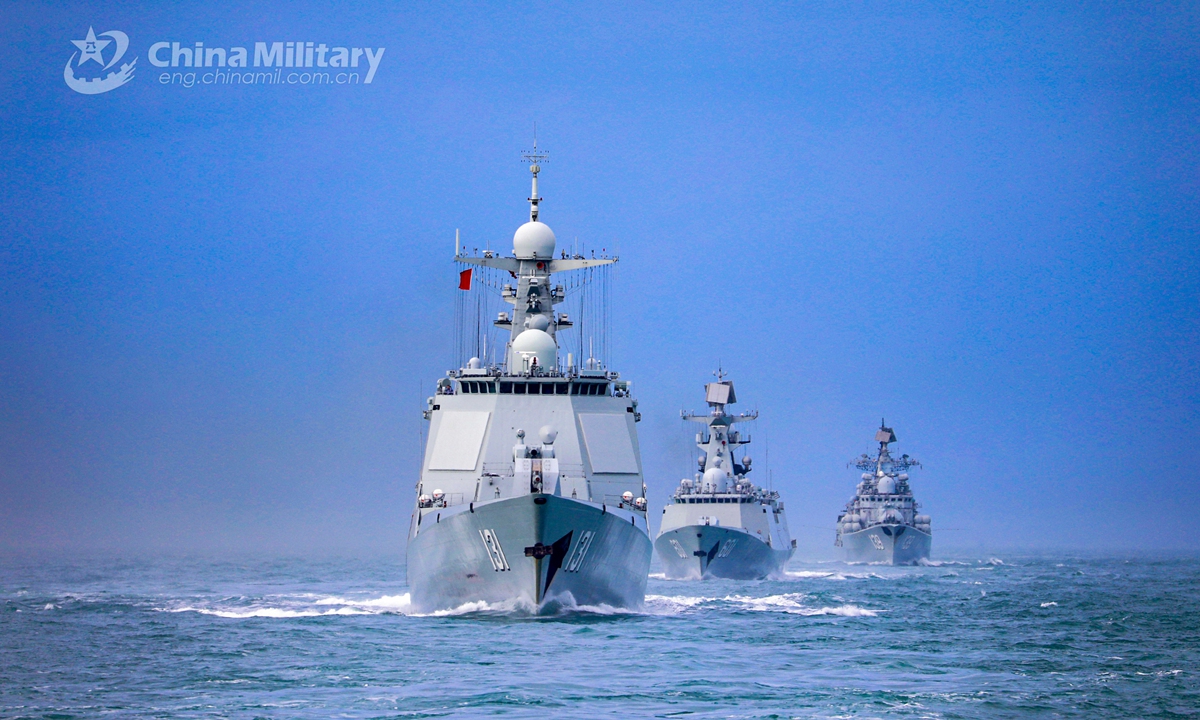The photograph captures three gray military ships navigating through a calm, blue ocean under a vibrant blue sky with hints of gray mist near the horizon. These ships are following each other in succession. The foremost ship, bearing the number 131 on both sides, features prominent control panels, radar domes, and various technical structures including square-shaped satellite equipment and cables. A red flag, presumed to be the Chinese flag, hangs from one of the cables. The two trailing ships, though similar in design, have numbers that are not entirely legible. Notably, in the upper left-hand corner of the image, there is a logo consisting of a star flanked by two half-circles, accompanied by the semi-transparent text "China Military" and the website "eng.chinamil.com.cn." This combination of shared descriptions provides a comprehensive and detailed view of the scene.